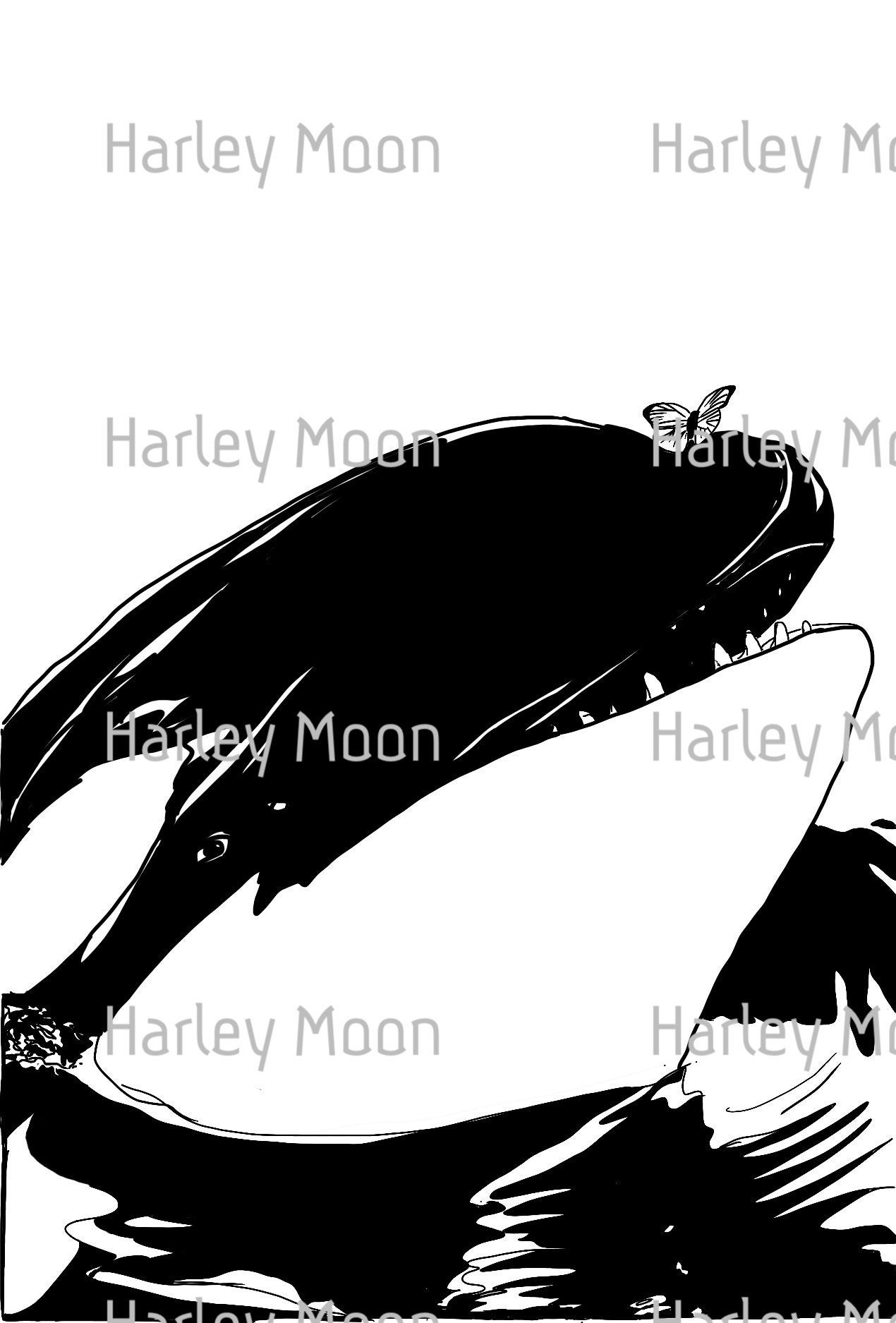This image is a detailed black and white illustration, predominantly featuring the head of a killer whale, reminiscent of the Shamu whale. The whale's head, marked by visible sharp teeth, is partially emerging from the water, and atop its nose rests a small butterfly. The background is stark white, offering a high contrast with the whale’s darker shading. Throughout the image, "Harley Moon" is written repeatedly in light gray or silvery text, giving the design a textured overlay. The photo is vertical and rectangular, emphasizing the striking presence of both the whale and the meticulously placed text.